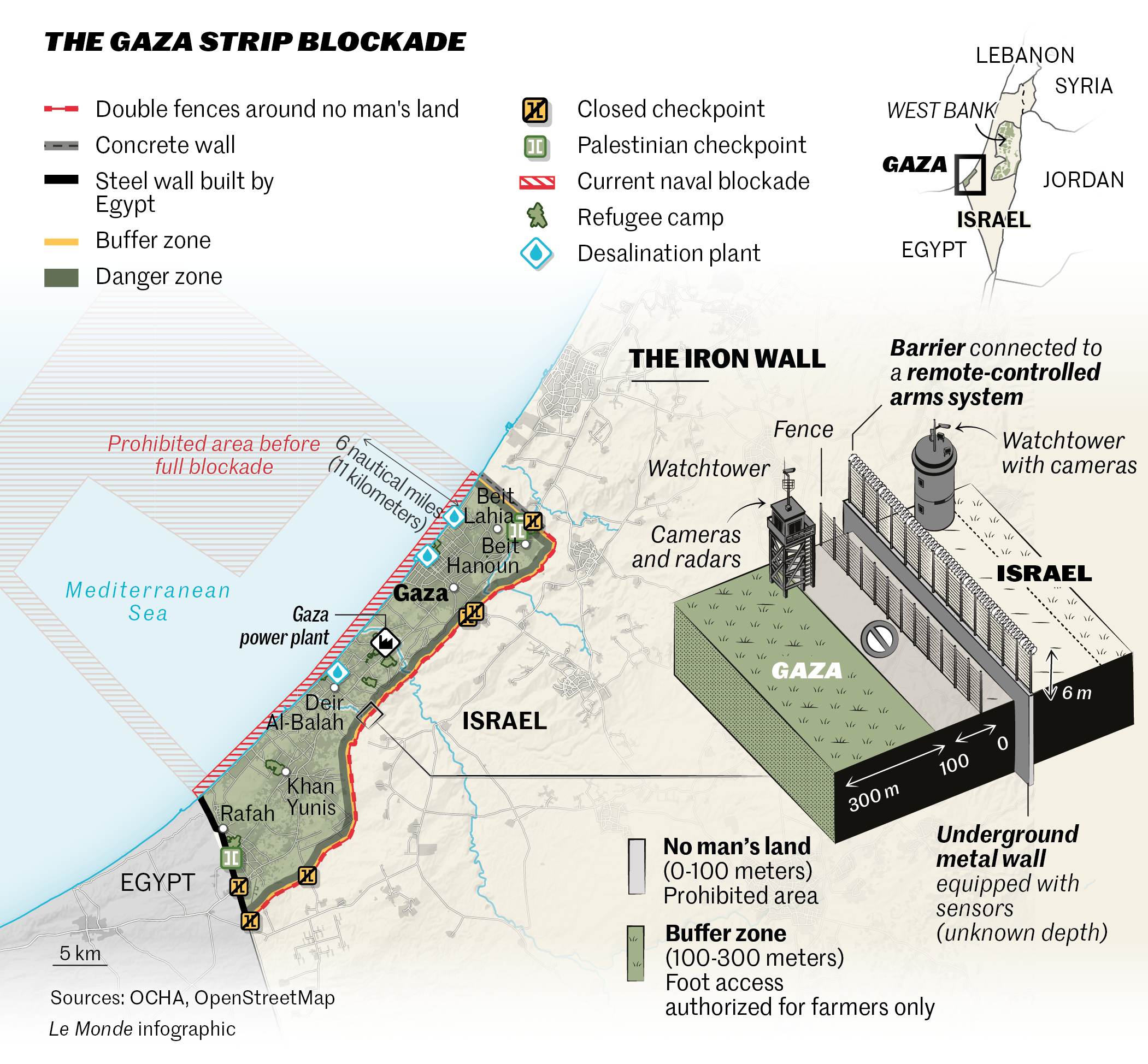A detailed map titled "The Gaza Strip Blockade" highlights the geopolitical boundaries of Gaza and its surrounding regions. The map prominently displays Israel to the right, the Mediterranean Sea to the left, and the northern tip of Egypt at the bottom. The main focus is on Gaza, which is marked in green, indicating a designated danger zone. 

A comprehensive legend at the top categorizes various elements, such as a red line marking double fences, a gray segment signifying a concrete wall, yellow denoting buffer zones, and green illustrating danger zones.

The map meticulously details numerous closed checkpoints along the border of Gaza. A zoomed-in section in the middle of Gaza's border reveals an area labeled "The Iron Wall," a formidable barrier integrated with a remote-controlled arms system. Additional symbols depict watchtowers flanking both sides of Gaza, with a fence running between them, emphasizing the heavily fortified nature of the region.